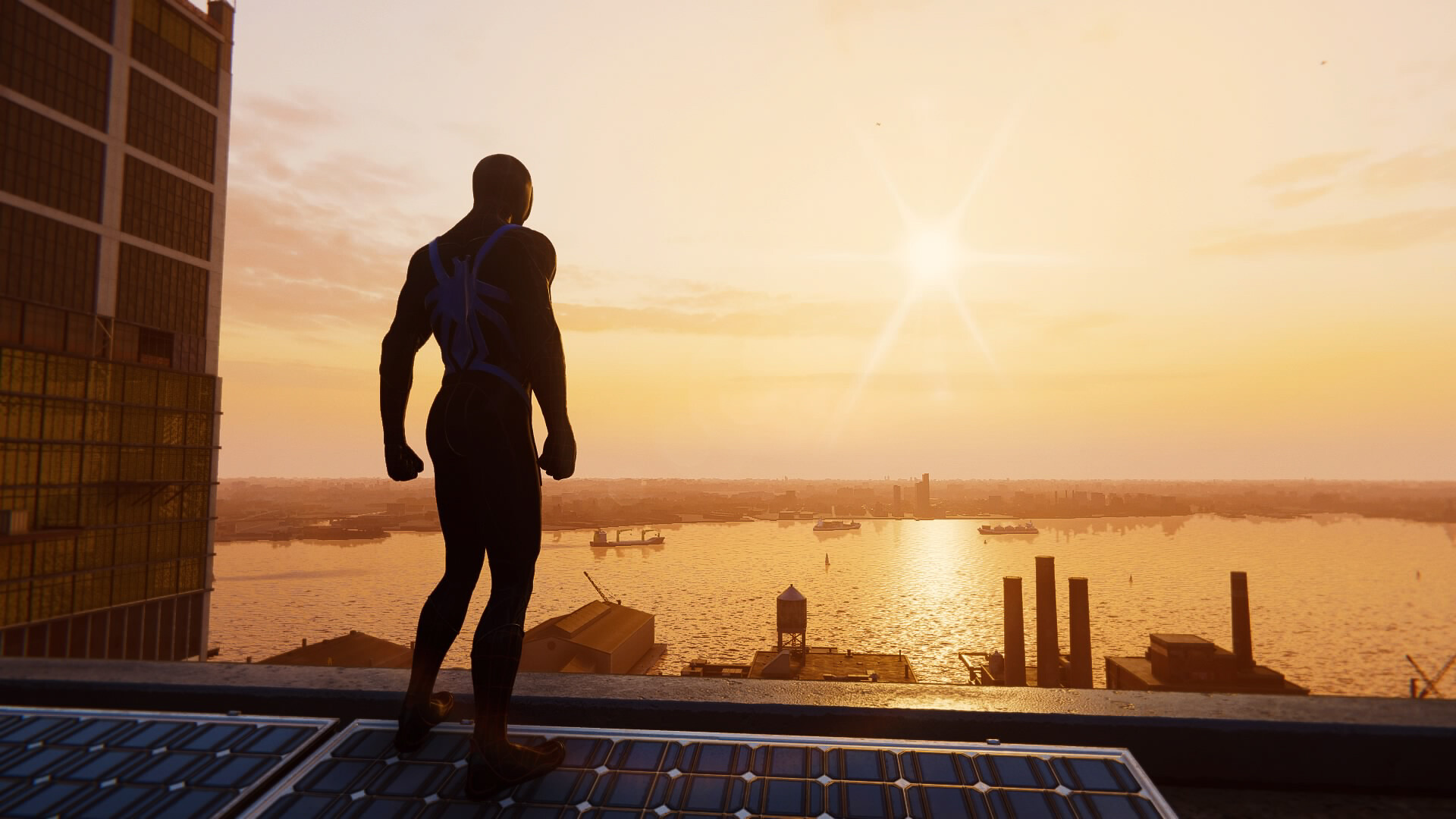The image showcases a meticulously detailed, amber-hued scene that exudes the complexity often attributed to AI-generated art. Dominating the foreground, a muscular, superhero-like humanoid figure stands poised on solar panels atop a rooftop. The figure’s rounded, masked face suggests a male presence, surveying the extensive industrial bay below. The landscape is dotted with chimneys, water towers, cranes, and warehouses, creating a busy, industrial atmosphere. 

Beyond the bay, the horizon is marked by a cityscape featuring high-rise buildings, with one prominent structure on the left. Approaching ships, equipped with oversized cranes and various items incongruously placed on their decks, populate the waters. Some buildings are reflected in the water below, while others curiously lack reflections, adding to the surreal quality of the scene.

The sun casts a dramatic glow through the clouds, illuminating the scene in a mix of black and amber. However, certain elements—like the disproportionate sizes of the ships and cranes, and the inconsistent reflections—reveal subtle anomalies. These peculiarities suggest the image might be an AI concept or a screenshot from a video game, as some details appear slightly off or out of place, enhancing the enigmatic nature of the composition.